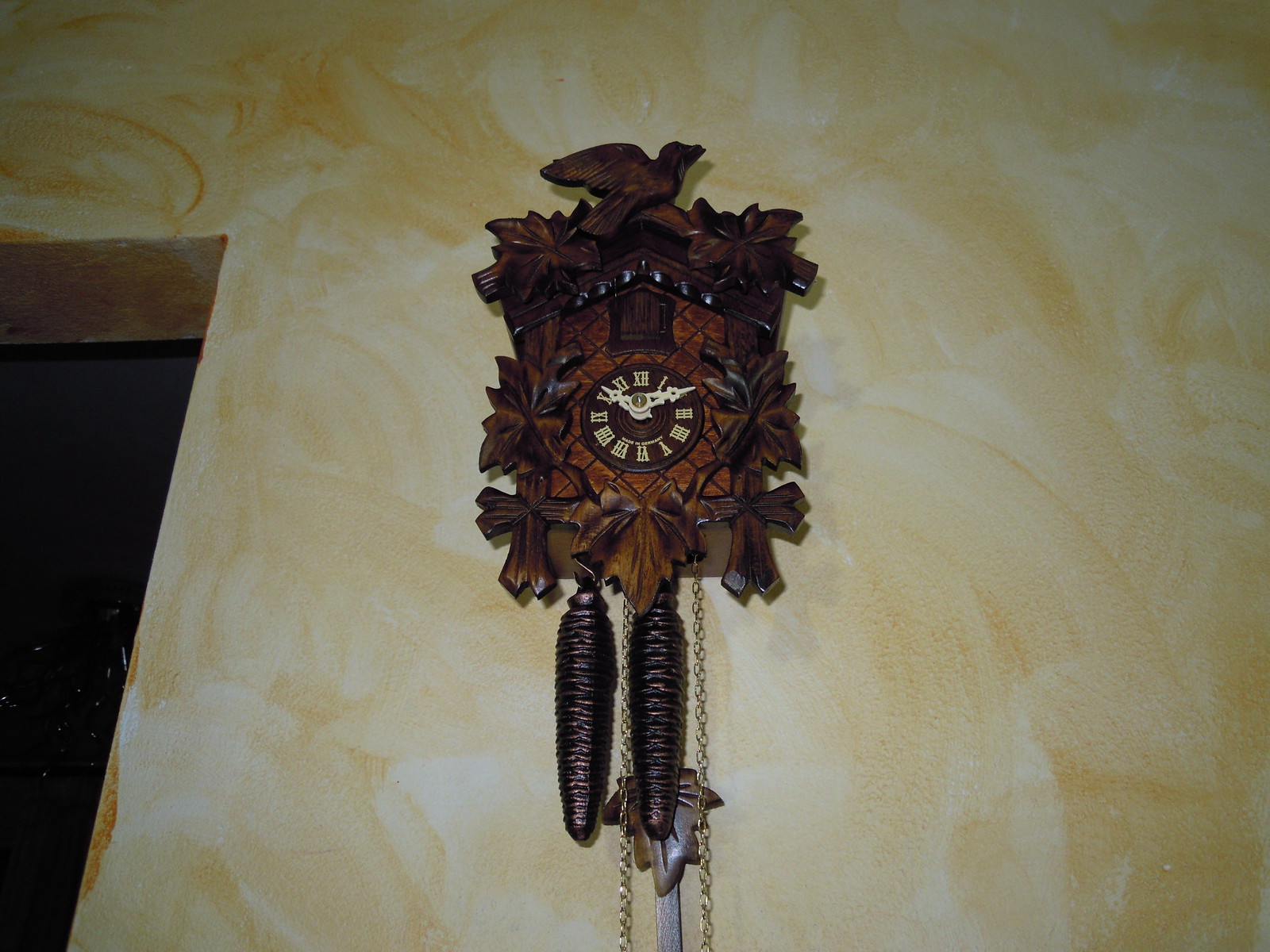A stunning high-quality photograph showcases an intricately carved wooden cuckoo clock mounted on a swirled design golden-yellow and white wall. The cuckoo clock's rich dark wood, tinged with subtle orangey tones, is adorned with a beautifully carved bird perched on the top. Flanking the clock face, ornate floral designs add an elegant touch, while a door with a crisscross pattern is positioned below them. The clock face itself, a deep chocolate brown, features off-white Roman numerals and matching hands, creating a striking contrast. Additional floral carvings embellish either side of the clock face, and the base displays two cross-like structures, complemented by a delicate leaf design. Suspended from the bottom are two slender, pine cone-shaped bronze weights, accompanied by a light brown leaf-like ornament. Two gleaming gold chains also dangle gracefully, completing the intricate and visually captivating design.